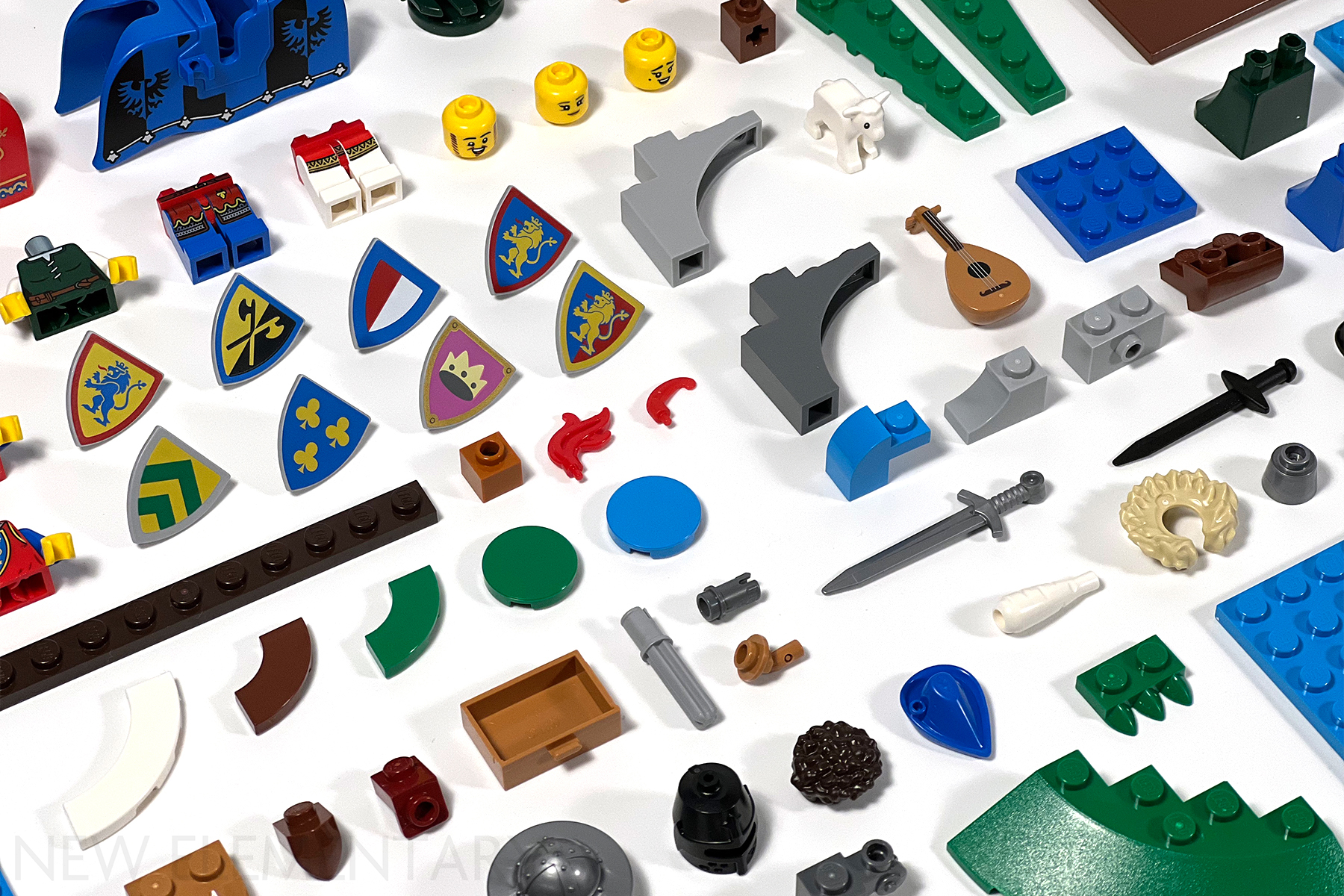This detailed image showcases an array of meticulously organized Lego pieces spread out on a white table, resembling a medieval-themed Lego set. The set includes various accessories and body parts, all neatly displayed. Visible are several yellow heads, blue torsos with yellow hands, legs, and numerous medieval weaponry such as swords and shields with distinctive emblems. Among the accessories, one can spot a brown guitar, possibly a ukulele, and several shields, some adorned with intricate illustrations. There are also pieces resembling a white lamb or a sheep, a cart or horse armor, and other miniature elements like staves and smaller armor pieces. The assortment is arranged systematically in rows, making it easy to distinguish. The background is white, indicating it could be taken indoors, and there is faint, barely legible writing in the lower left-hand corner that appears to say "New F-L-E-M-A-N-T-A-R" in light gray font. The overall scene conveys a rich variety of Lego parts in colors such as blue, yellow, green, black, and gray, all contributing to the medieval aesthetic of the set.